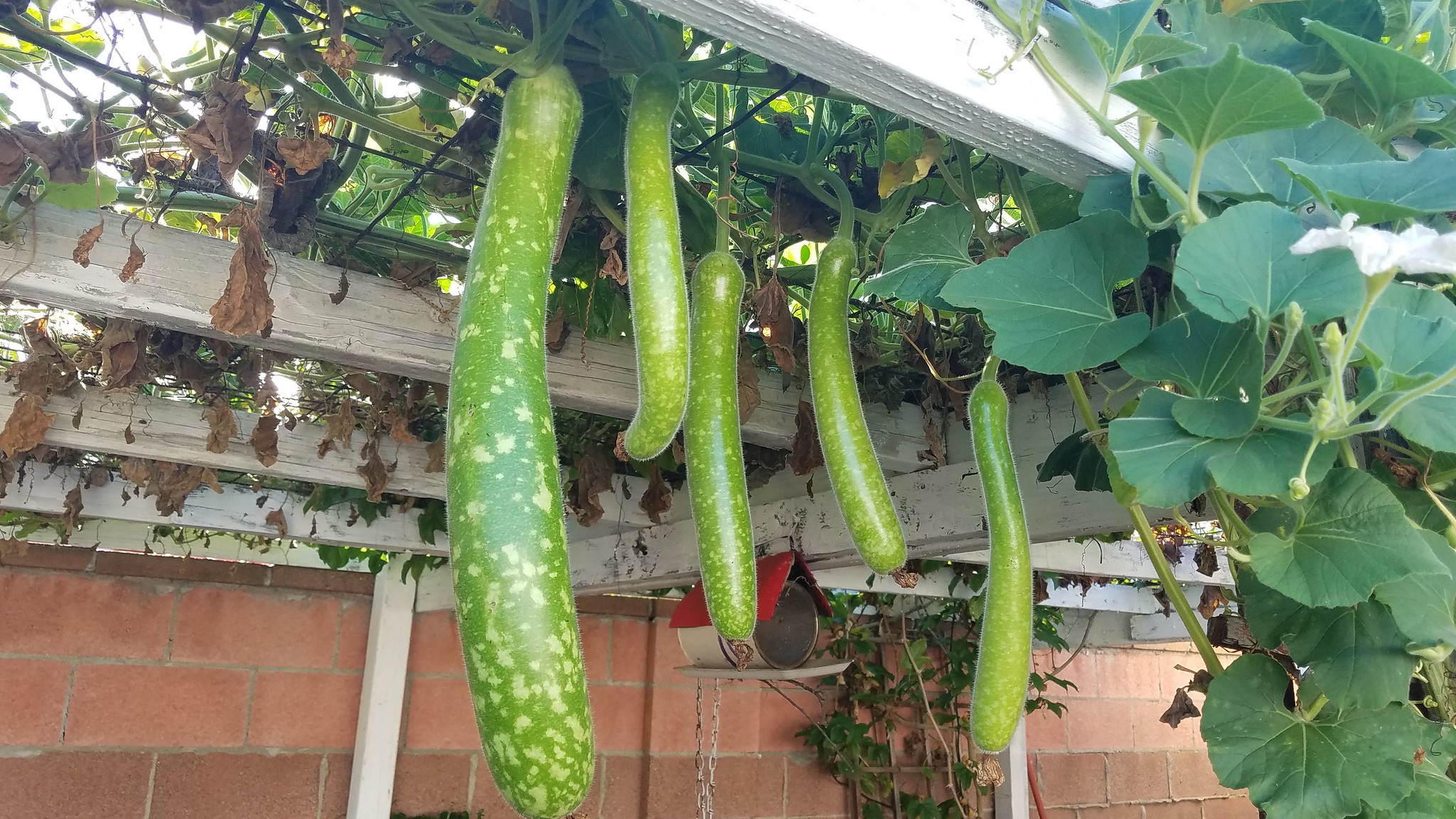The image showcases a ceiling made out of a wooden structure, adorned with a mix of vibrant and withered foliage. On the right side, large, vivid green leaves with long stems cascade down, while on the left, the leaves appear withered, brown, and crumpled, resembling pieces of paper. In the center, long, curved green vegetables, similar to zucchinis with yellow spots, hang down. Below this greenery is a light brown brick wall, suggesting an enclosed garden space. Additionally, a white fence, partially covered with ivy and extended by an overhead structure, supports the plants. A tin can with a red roof—resembling a birdhouse—hangs centrally, adding a quaint touch to the scene.